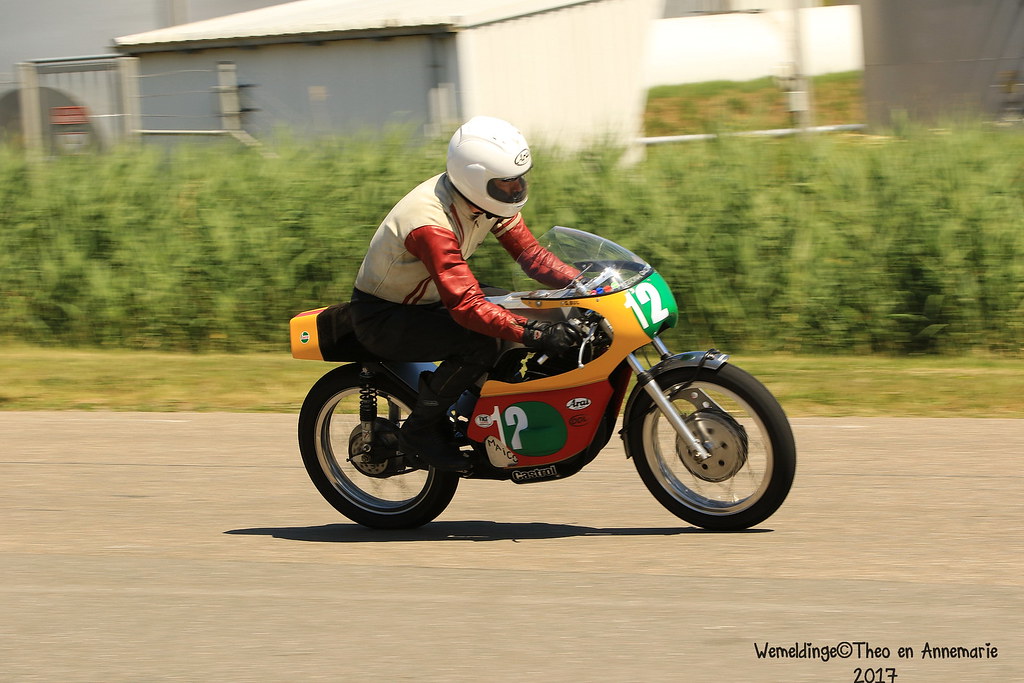In this image, we see a motorcyclist riding his bike along a gray asphalt road, positioned directly in the center of the frame. The motorcyclist is fully geared up, featuring a white helmet, a jacket with red sleeves and a white body, and dark-colored pants. His motorcycle stands out with distinctive red, yellow, and green livery, prominently displaying the number 12 on both the front and sides.

The scene is set outdoors during the day, likely on the side of a highway. In the immediate background, there's a strip of grass bordered by some bushes. Further back, partially blurred, we can discern several buildings and gates. One of these structures appears to be a large building with a blue and white facade. The text in the bottom right corner reads "We Meldage Theo and Anne Marie 2017," suggesting a possible copyright statement. The predominant colors in the image include gray, black, silver, red, yellow, green, white, off-white, and light blue.